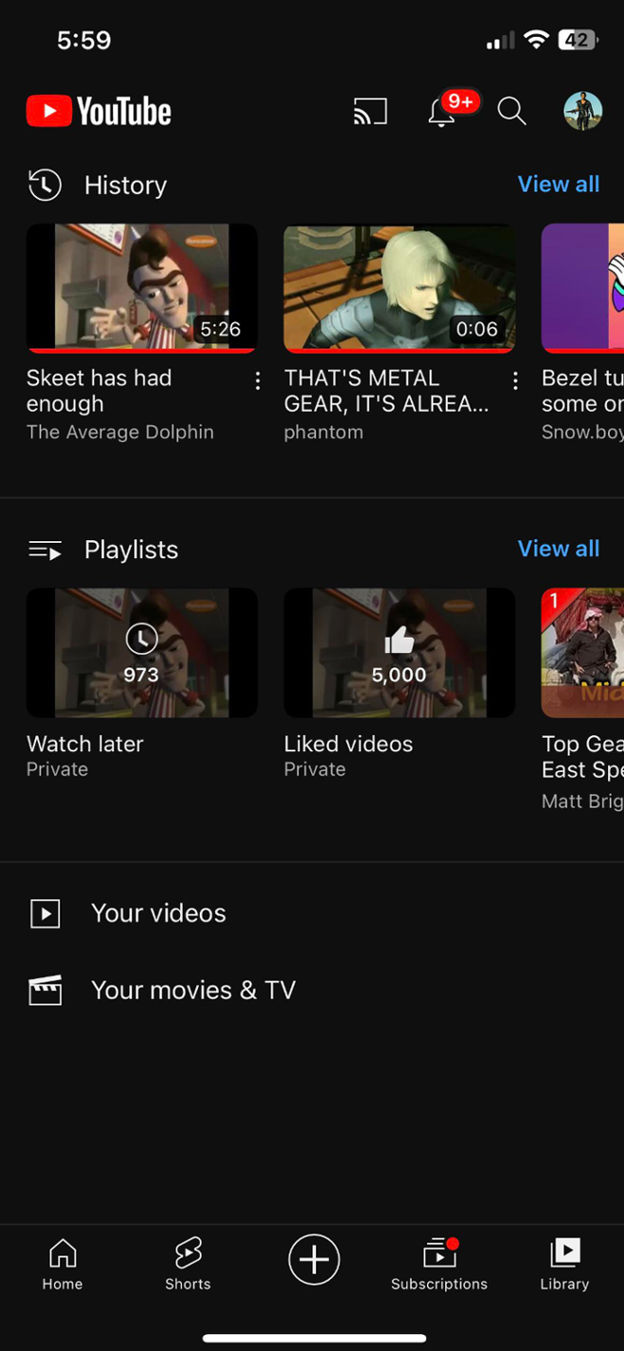This image is a screenshot of a YouTube webpage displayed on a mobile device. The background is solid black. 

- **Upper-Left Corner:** In white text, the time is displayed as "5:59."
- **Upper-Right Corner:** There are two out of four Wi-Fi bars, Wi-Fi is enabled, and the battery icon shows a 42% charge remaining.
  
**YouTube Interface Details:**

- **Below the Time:** The YouTube icon is present—a red box with a play button and "YouTube" written in white next to it.
- **Text Sections:**
  - Beneath the YouTube icon, "History" is written in white text.
  - Below "History," there is an image thumbnail of a video featuring a cartoon character. The video's duration is 5 minutes and 26 seconds, and the title reads "Skeet has had enough. The average dolphin."
  - To the right of the video thumbnail, there is an image that appears to represent a gaming character from Metal Gear Phantom, and the timestamp shows ".06 seconds."
  - Below this area, there is a section for a playlist labeled "Watch Later" with a privacy setting denoted as "private."